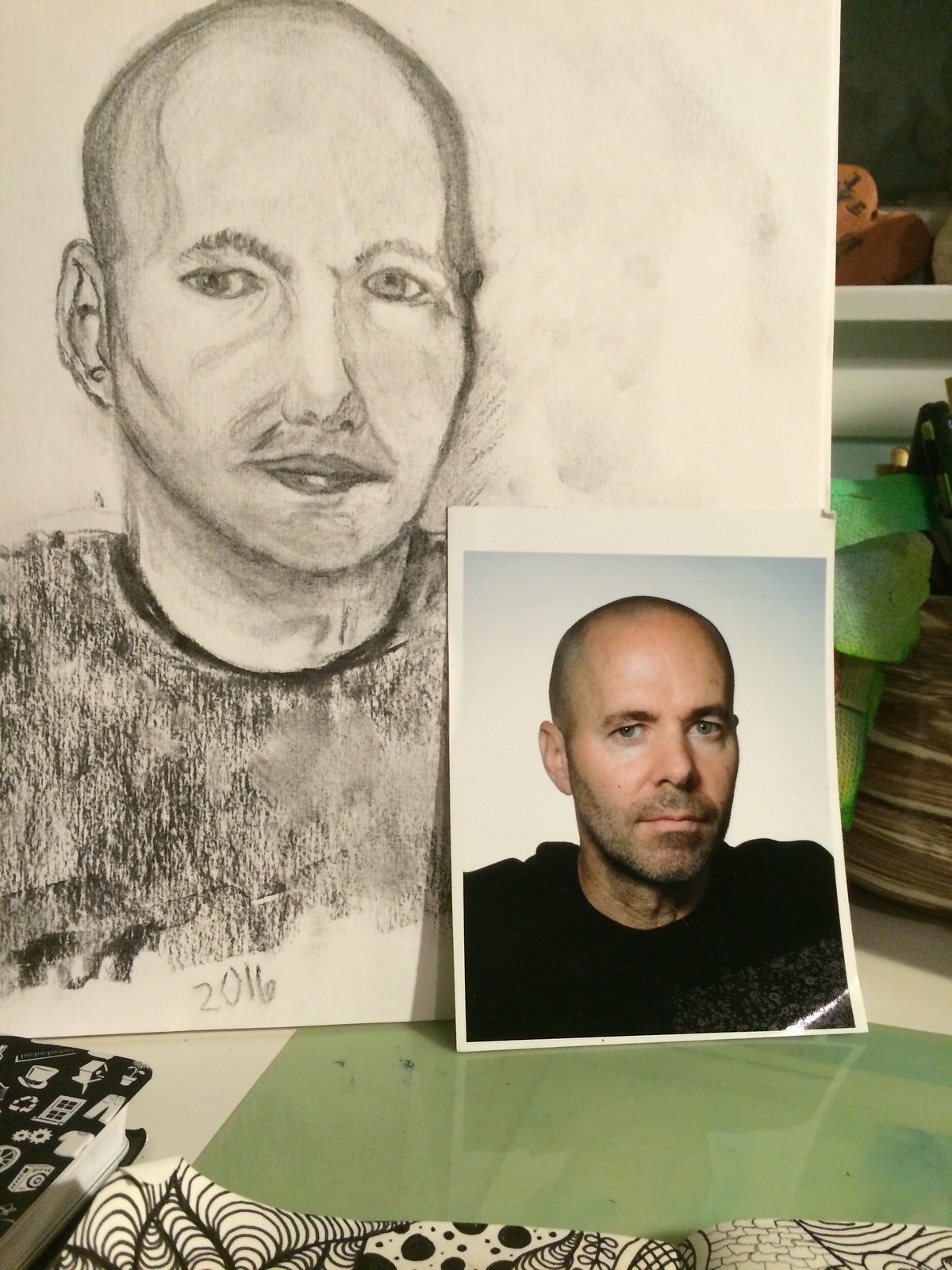This image features a detailed pencil sketch of a photograph, prominently displayed against an off-white background. The sketch portrays a mostly bald man, facing the camera to reveal the front of his face and one ear, mirroring the pose from the original photograph. The man, depicted with a shaved head and a notable five o'clock shadow, wears a dark shirt in both representations. The original photograph had a light blue background, but in the sketch, the background is left blank to highlight the subject. Notably, the bottom of the pencil drawing is marked with the year "2016."